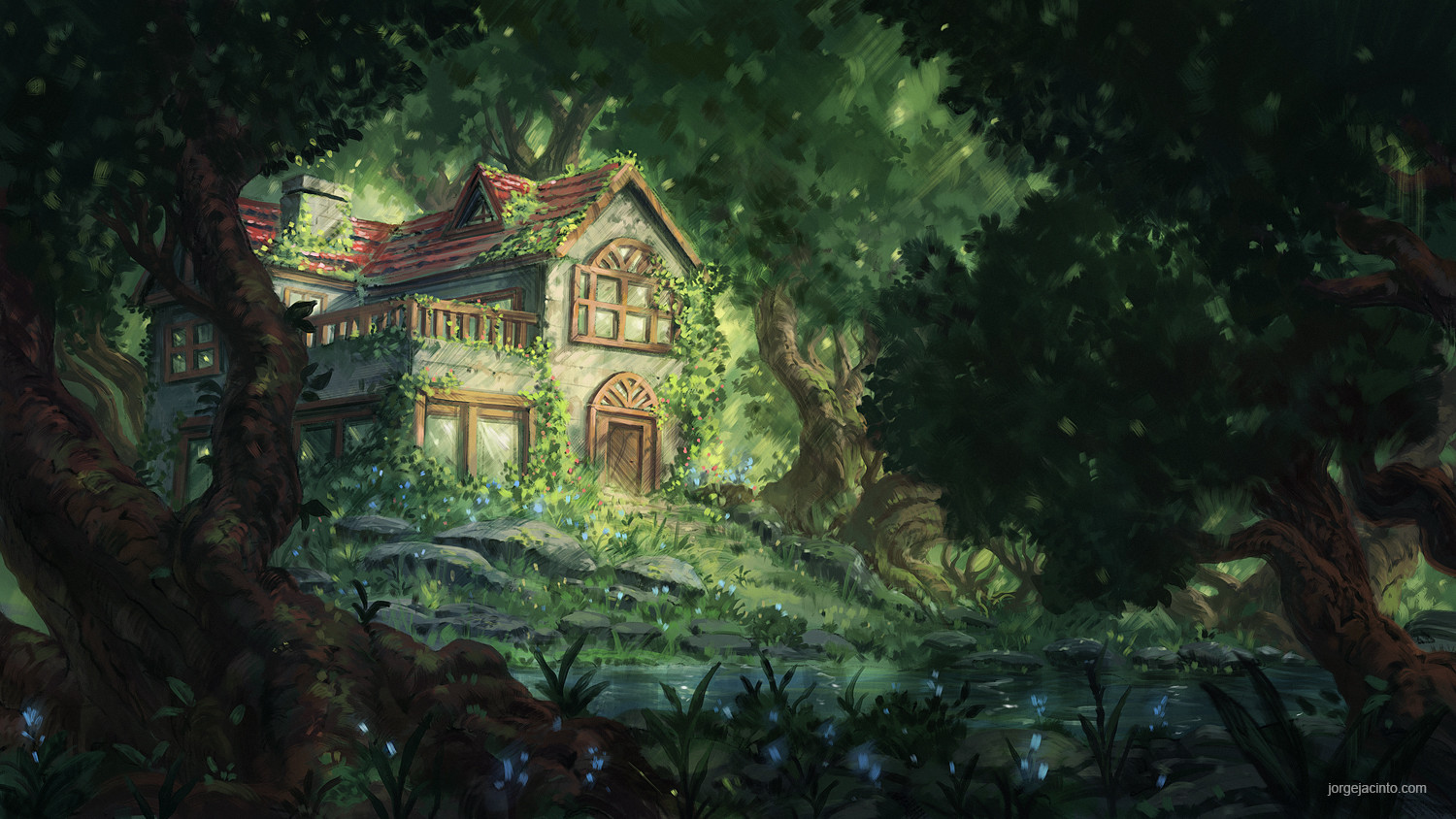The image portrays a meticulously drawn painting of a serene woodland scene, centered around a slightly aged, yet well-maintained, two-story house with an attic. The house, resting on a small hill, features a reddish shingle roof, a wooden front door, and a quaint balcony or porch on the upper story. Its gray and brown exterior is adorned with ivy and green leaves creeping up the sides, adding to its rustic charm. The foreground is dense with trees that possess thick green foliage and brown trunks, creating a lush, verdant environment typical of a jungle. A gentle stream flows in front of the house, accompanied by small blue flowers dotting the landscape. The overall ambiance suggests nighttime, as there is no visible sunshine, yet the house remains well-illuminated. The bottom right corner of the painting is marked with the artist's watermark, "jorgejacinto.com".